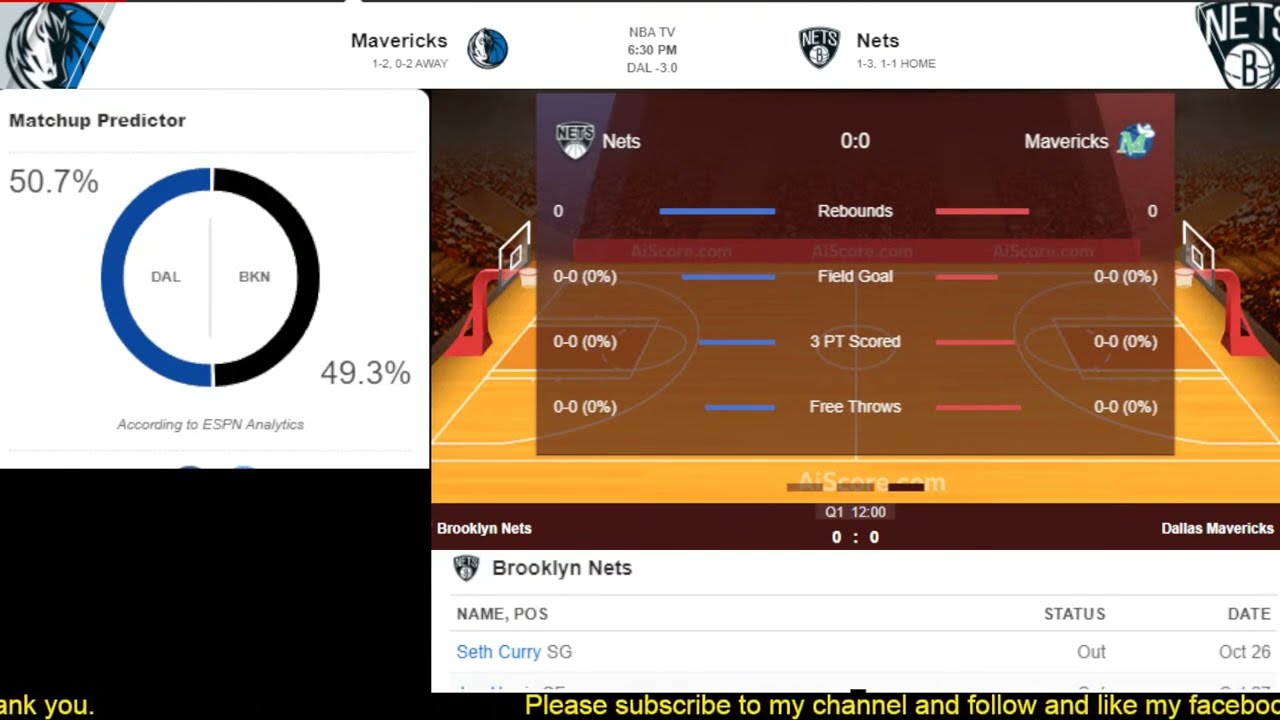The image is a detailed screenshot from a sports website comparing the Brooklyn Nets and the Dallas Mavericks in an upcoming basketball game. In the middle of the image, there is a central square shadowed over the background. The upper left corner of this square features the word "Nets" in black text with a green outline, accompanied by the Nets' logo. The upper right corner shows "Mavericks" with their logo, a green-colored 'M' encircled by blue. Prominently in the center of the square, the score is displayed as "0:0," indicating the game has not yet started. Below this are four lines of statistics in white text: rebounds, field goals, three-point scoring, and free throws, each accompanied by blue and red lines to show team scores and percentages.

The background reveals a semi-transparent, simulated basketball court with a yellow surface and white lines. The court features clear acrylic backboards with white outlines and orange supports. Above the main square, there's a white bar displaying "NVATV 6:30 PM DAL-3.0" in the center, flanked by "Mavericks" on the left and "Nets" on the right. Additional team records are shown below each name: Mavericks at 1-2 and 0-2 away, Nets at 1-3 and 1-1 home. 

On the far left is a white square labeled "Matchup Predictor" in black text, with a circle split into two colors – blue and black. It forecasts a 50.7% chance for the Mavericks (DAL) and a 49.3% chance for the Nets (BKN), according to ESPN analytics.

The bottom of the screenshot includes a black bar with yellow text, urging viewers to "please subscribe to my channel and follow and like my Facebook." Above this bar, a centered white section provides player status updates: it lists "Brooklyn Nets" at the top, with player details below, including "Seth Curry SG, Out, October 26th."

Overall, this image combines rich visual and textual information to present a comprehensive breakdown of the anticipated game between the Nets and the Mavericks, enriched with statistics, team logos, player statuses, and viewer engagement prompts.